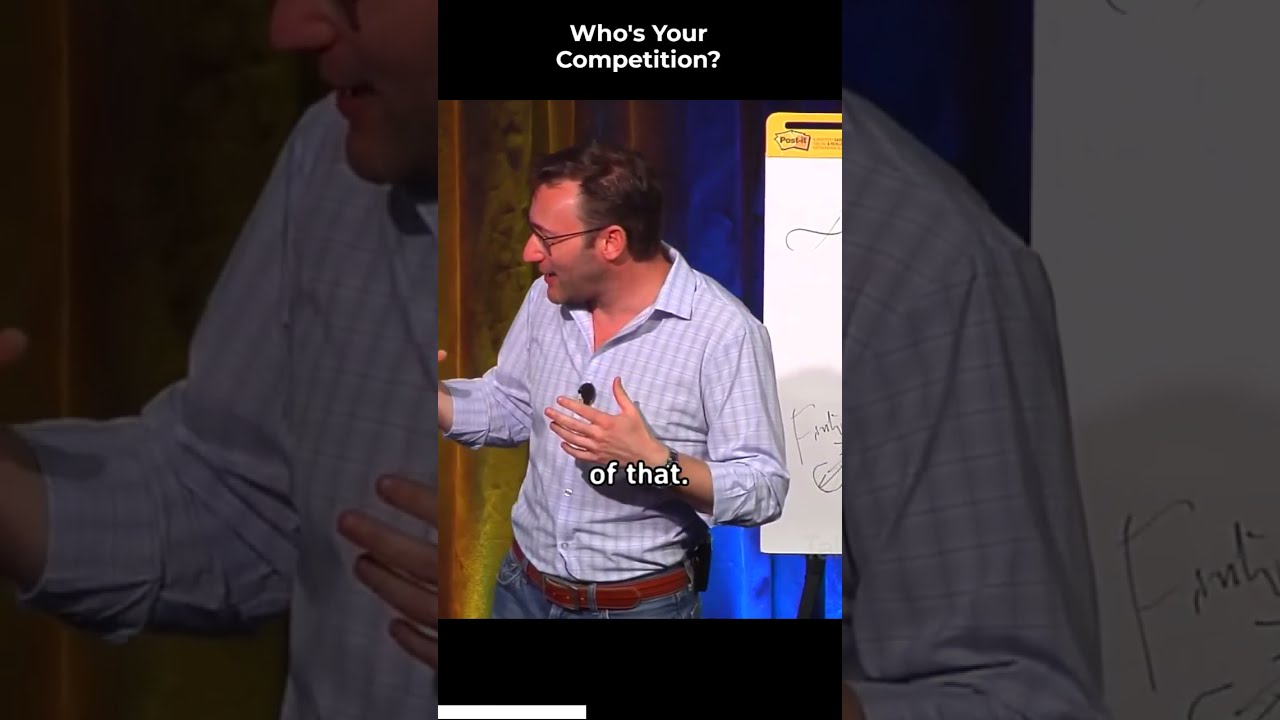The image is a screen grab from a vertical TikTok or social media video featuring a mid-40s Caucasian man with short brown hair and glasses. He has a slight 5 o'clock shadow and is partially balding. He's wearing a white and blue striped button-up shirt, blue jeans with a brown leather belt, and a black watch on his wrist. The man appears to be making a presentation, indicated by the microphone on his lapel and his outstretched arms as if explaining something. He stands before a colorful background that suggests a stage or backdrop, although the specifics are out of frame. Behind him is a whiteboard or post-it board with some visible letters, such as an 'F'. The image has black borders at the top and bottom, giving it a framed appearance. The top of the image contains white text reading, "Who's your competition?" and the middle section has the subtitle "Of that period," capturing the man mid-sentence. The background also includes a blown-up close-up of his face, shirt, hands, and part of the board he's standing in front of.